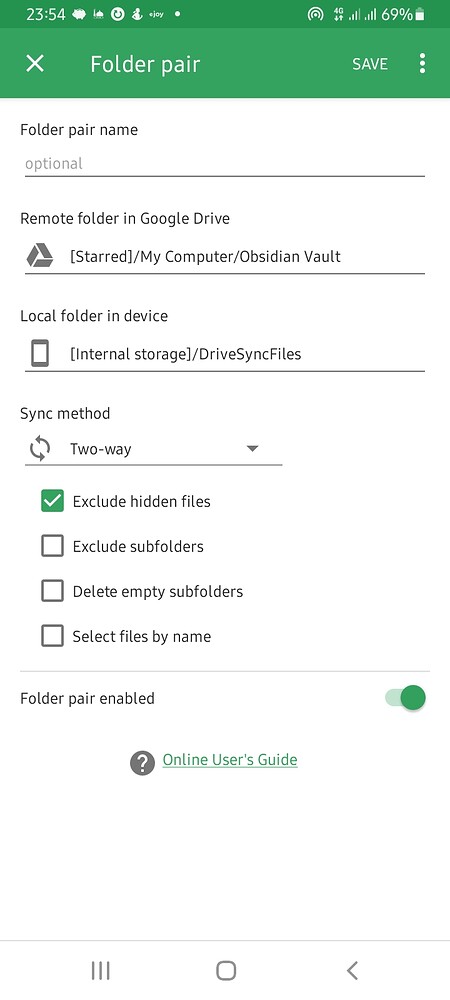The image displays a cell phone screen with various settings and information. 

1. **Top Section**: 
   - A green strip is present at the top of the screen.
   - The upper left corner shows a timestamp: "23:54".
   - A series of mostly unrecognized icons are displayed, including one indicating "rotate" and another on the right side symbolizing data sharing.
   - The screen shows connectivity with cell signal bars and a battery level at "69%".

2. **Header Section**:
   - The left side features an "X" icon.
   - Centrally located is the text "Folded Pair".
   - On the right, there is a "Save" option accompanied by a vertical ellipsis (three dots).

3. **Main Interface**:
   - **Folded Pair Name**: Displayed on a white background with a gray placeholder text "Optional".
   - **Remote Folder**: Specifies "Google Drive".
   - A list under "Remote Folder" includes "Starred", "My Computer", and "Obsidian Vault", separated by a line.

4. **Local Folder Section**:
   - Displays options such as "Device", "Internal Storage", and "Drive Sync Files", with an unchecked box in front.
   - This section is also separated by a line.

5. **Sync Settings**:
   - Includes settings for "Sync Method" with a drop-down menu showing "Two Way".
   - Checkboxes for options like "Exclude Hidden Files" (checked), "Exclude Subfolders", "Delete Empty Folders", and "Select Files by Name".

6. **Additional Information**:
   - Text indicating "Folded Pair Enabled" next to a question mark icon in a gray circle.
   - "Online User's Guide" is displayed in green text, underlined, next to a green toggle switch, indicating it is enabled.

This detailed description ensures that every element and textual information displayed on the cell phone’s screen is adequately captured and clearly presented.